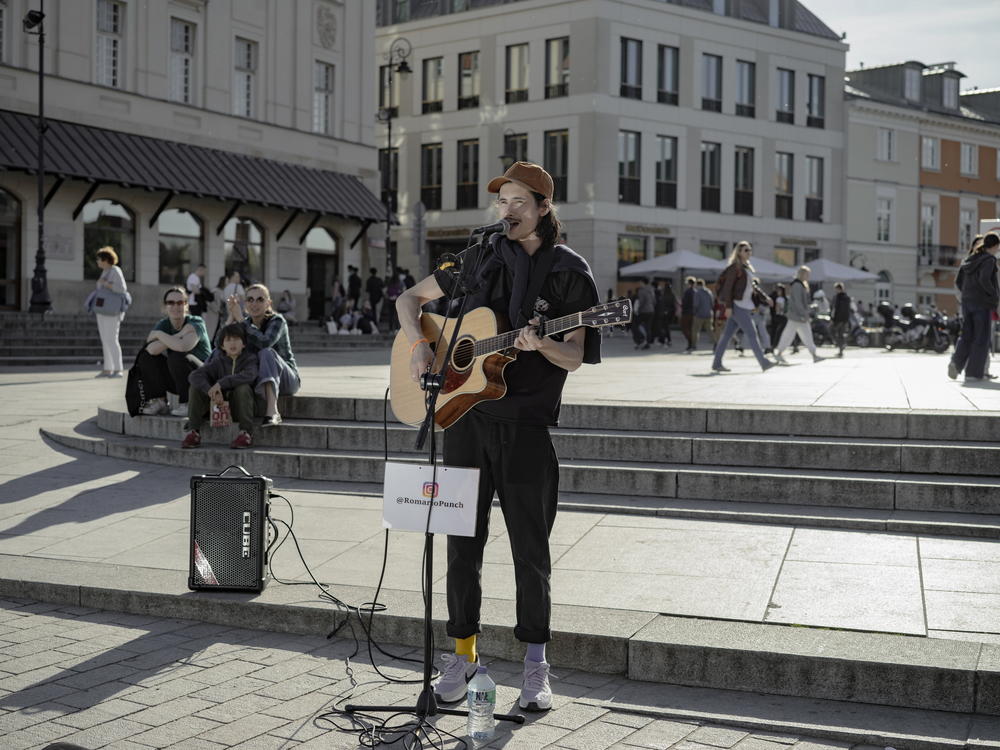In a bustling city plaza with brick pavement and a three-row flight of concrete steps, a man performs as a busker. He's positioned at the bottom of the stairs, standing in front of a microphone stand and singing while playing an acoustic guitar. He wears a dark short-sleeved T-shirt, dark pants, white tennis shoes, and a brown baseball cap. Over his shoulders is a black sweater tied in the front. Notably, he sports mismatched socks—a grey one on his left leg and a yellow one on his right leg, along with an orange wristband on his right arm. A white piece of paper taped to the microphone stand features the Instagram logo and the handle @RomarioPunch. To the left of the performer is a rectangular box-shaped speaker. Behind the speaker, two women and a boy sit on the steps, captivated by the music. In the background, people in long coats and pants walk by, and the scene is framed by tall buildings in shades of white, grey, orange, and cream, some with tall windows and others with small ones. The lively setting captures a snapshot of urban life interspersed with moments of musical enjoyment.